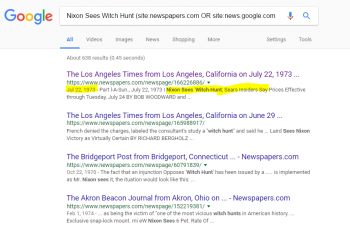In the image, a Google search page is prominently displayed. In the top left corner, the iconic multicolored Google logo is visible. Below the logo is the search bar, which contains the query "Nixon sees witch hunt. Site: newspapers.com" or "Site: news.google.com". Beneath the search bar, the standard selection of Google search options is shown, including tabs for All, Videos, Images, News, Shopping, and More. Also present are buttons for Settings and Tools.

The search results section shows several articles. The first article is titled "The Los Angeles Times from Los Angeles, California, on July 22, 1973," sourced from newspapers.com. The smaller text under the title of this article is blurred and illegible. The second article is "The Los Angeles Times from Los Angeles, California, on June 29th," though the specific year is not evident. Further down, another result titled "The Bridgeport Post from Bridgeport, Connecticut," also sourced from newspapers.com, is displayed. The final visible search result is from the "Akron Beacon Journal from Akron, Ohio." 

Each article snippet indicates the source and location, providing a historical context to the search query related to Nixon, presumably referencing events during the Watergate scandal era.